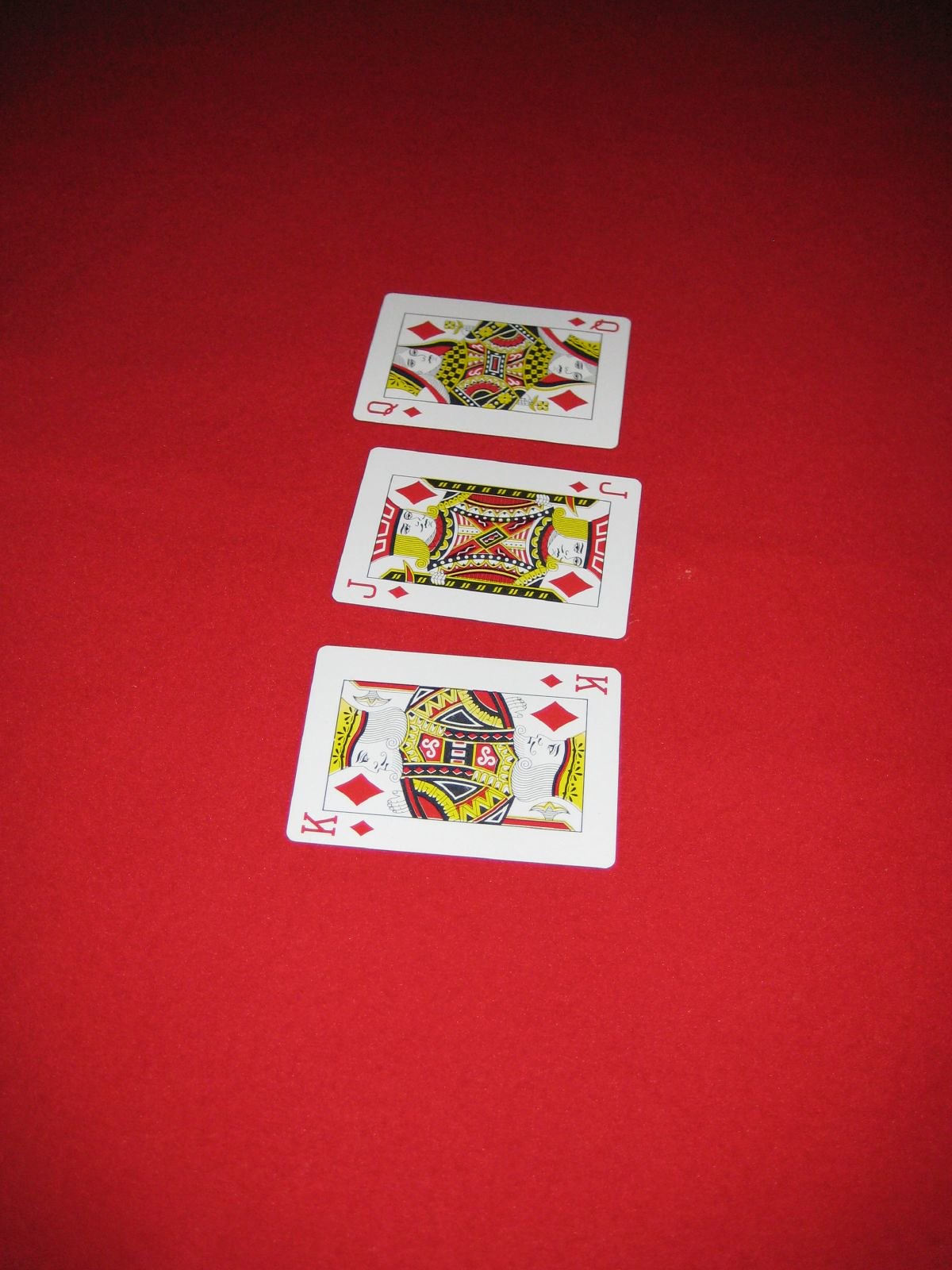This long-form photograph features a rich, possibly velvet, red tablecloth as its backdrop. At the center of the image, three playing cards are prominently displayed in a linear arrangement: the Queen of Diamonds, the Jack of Diamonds, and the King of Diamonds. The Queen is positioned closest to the viewer, partially overlapping the Jack, which in turn overlaps the King. Noticeably, the Queen and Jack face left, while the King looks to the right. The surrounding areas of the photograph are bathed in darker shadows, emphasizing the central alignment of the cards, which are illuminated as though by an unseen spotlight. No other elements are visible in the frame, keeping the focus solely on the cards against the opulent red cloth.